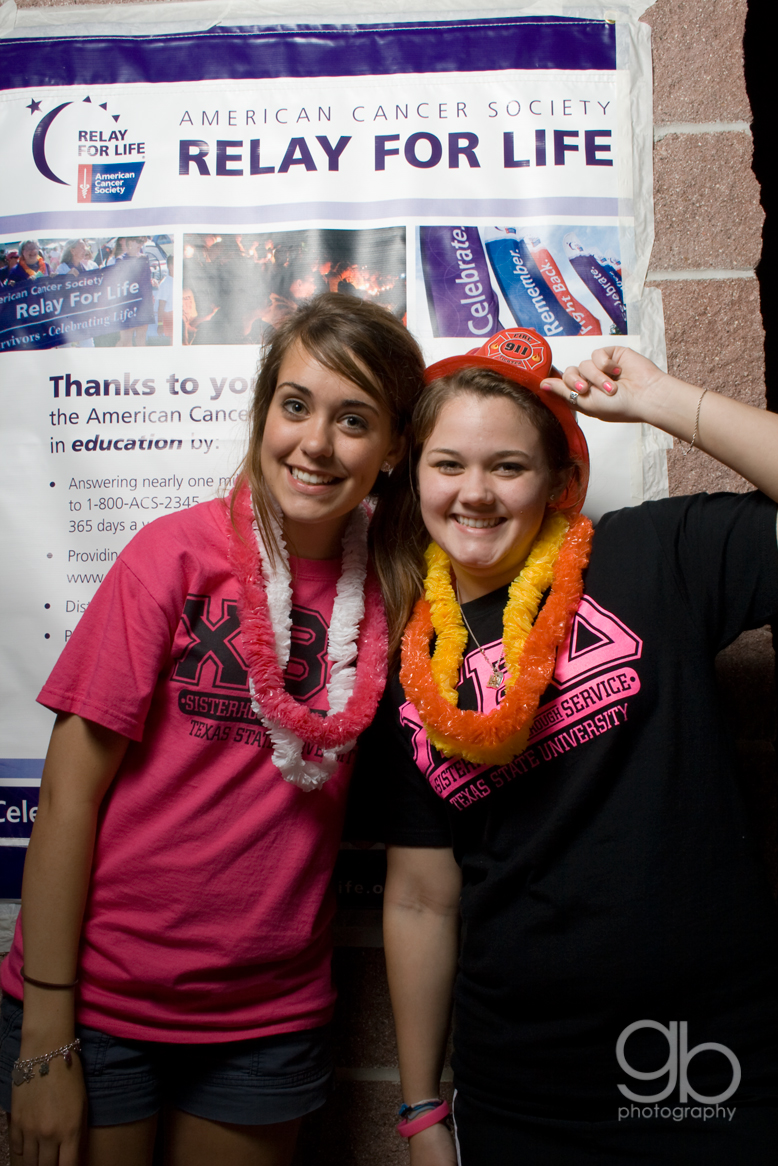In this image captured by GB Photography, we see two young women, presumably college students from Texas State University, sitting against a brick wall. Both are smiling warmly, exuding a sense of camaraderie and joy. The woman on the left has medium-length brown hair and is wearing a pink shirt bearing the words "Texas State University Sisterhood," paired with blue jean shorts. She has two plastic lace necklaces – one white and one pink – along with bracelets, including a charm bracelet.

The woman on the right is wearing a black t-shirt with pink lettering that also states "Texas State University." She sports a red 9-1-1 firefighter hat, which she touches with her left hand. Around her neck are two plastic lace necklaces in shades of yellow and orange, and she has several gel bracelets and a ring on her beautifully painted hand.

In the background, a large banner prominently displays "Relay for Life" and the "American Cancer Society" logo, hinting that the scene might be part of a charitable event. The GB Photography logo is seen in the bottom right corner of the image.